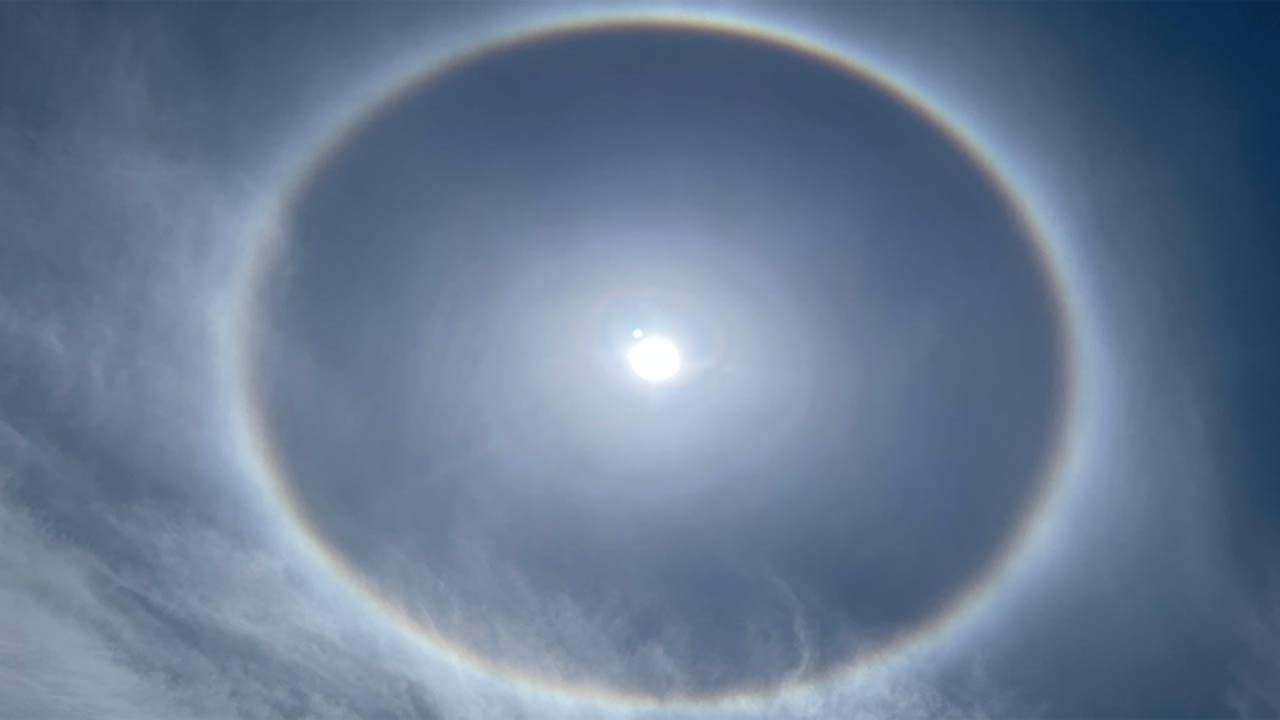The image depicts a dramatic eclipse in the sky, captured in landscape mode. The background features a blend of deep blue and dark gray, with wisps of clouds adding a misty, ethereal quality. At the center, a bright, perfectly circular burst of light marks the sun being partially obscured, potentially by the moon. Concentric rings of glowing light radiate outward from this central bright spot, creating a striking halo effect. Surrounding this luminous core is a large, dark blue circle, which is further enclosed by a thin brown stripe and a larger white halo. The intricate pattern of light and shadow, with its peaceful, atmospheric wisps, emphasizes the serene yet awe-inspiring nature of the eclipse.